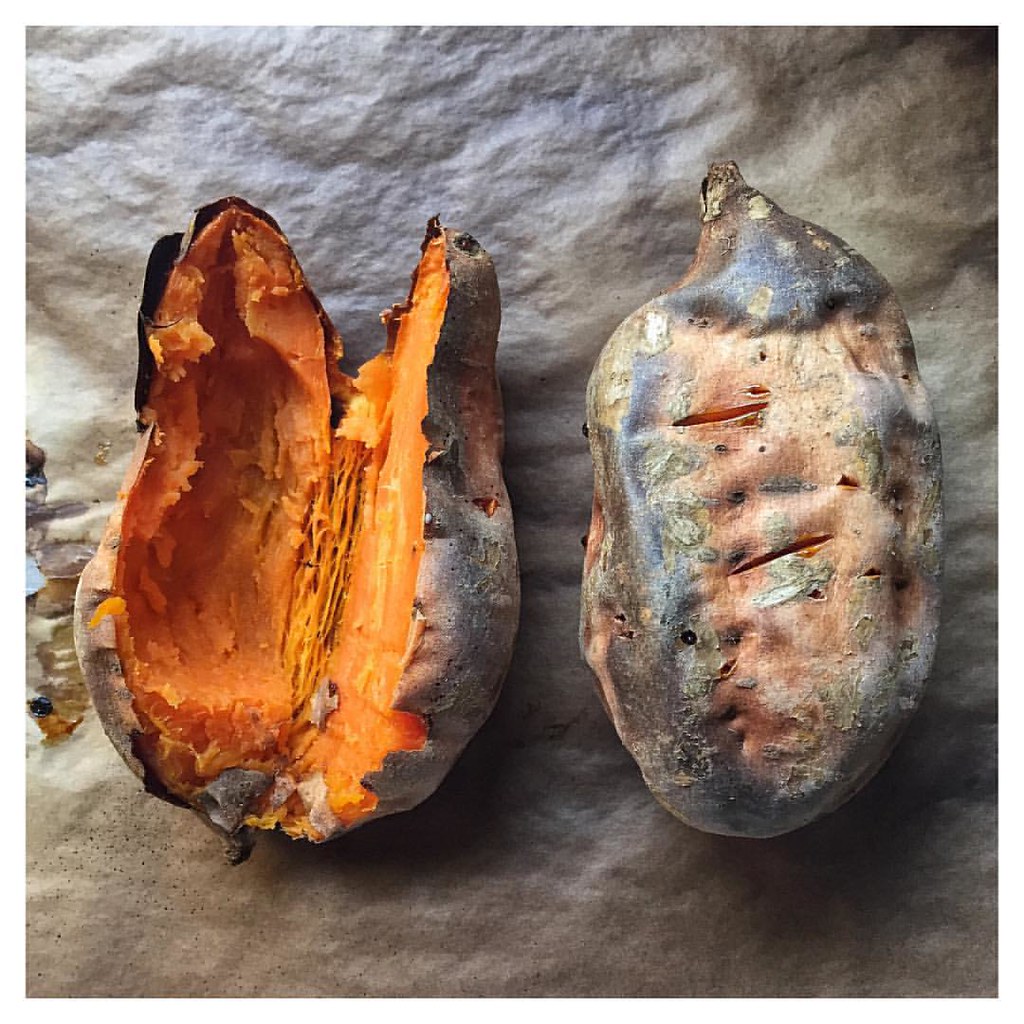This image captures a pair of baked sweet potatoes resting on a dark, burnt parchment paper background. Both sweet potatoes have their skins on, showcasing distinctive preparations. The sweet potato on the left is cut open, revealing its vibrant orange flesh. Part of the interior has been scooped out, indicating it was sampled. Meanwhile, the sweet potato on the right remains whole, displaying evident knife stabs used for steam release during baking. Its skin appears blackened and dry, suggesting it’s been sitting out for a while. The contrast in textures and conditions highlights the natural beauty and versatility of baked sweet potatoes.